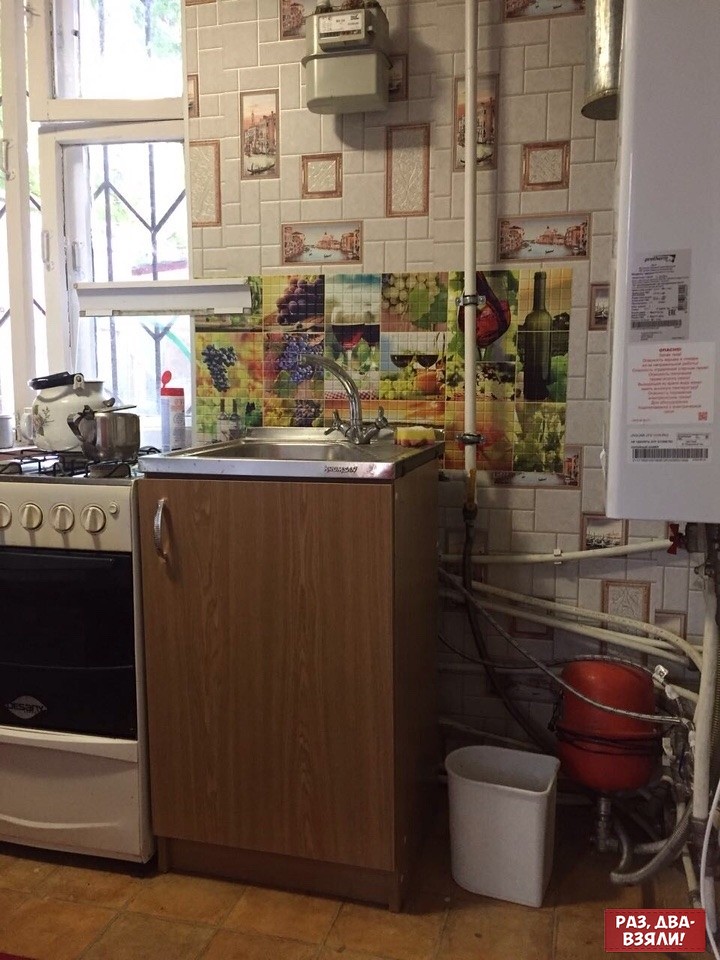This photograph captures a small kitchen featuring a comprehensive view of one wall. Dominating the left side of the image is a white and black stove with visible four knobs, a glass window in the oven door, and a leaf-shaped logo beneath. The stovetop hosts two kettles: a white one with a black handle and a silver one with a silver handle and black spout. Adjacent to the stove, a brown wooden cabinet supports a stainless steel sink with a curved faucet and dual three-knob handles. A small cylindrical item, likely soap, is positioned beside the faucet. Above the sink, a series of decorative tiles form a striking backsplash showcasing scenes of wine, grapes, and old cities like Venice within a collage pattern. 

A window with white frames and black wrought iron bars adorns the wall behind the stove. Above the sink, an electric reading meter box is affixed. Completing the right side of the kitchen setup is a comprehensive hot water system, which includes a white heater mounted on the wall and a red pressure tank connected by various pipes. Between the sink cabinet and the red tank is a rectangular white wastebasket with a rounded edge. A silver canister appears in the upper right corner of the photo, alongside a red rectangular label emblazoned with Cyrillic text. The kitchen floor is a warm terracotta tile, providing a cohesive look to the compact space.